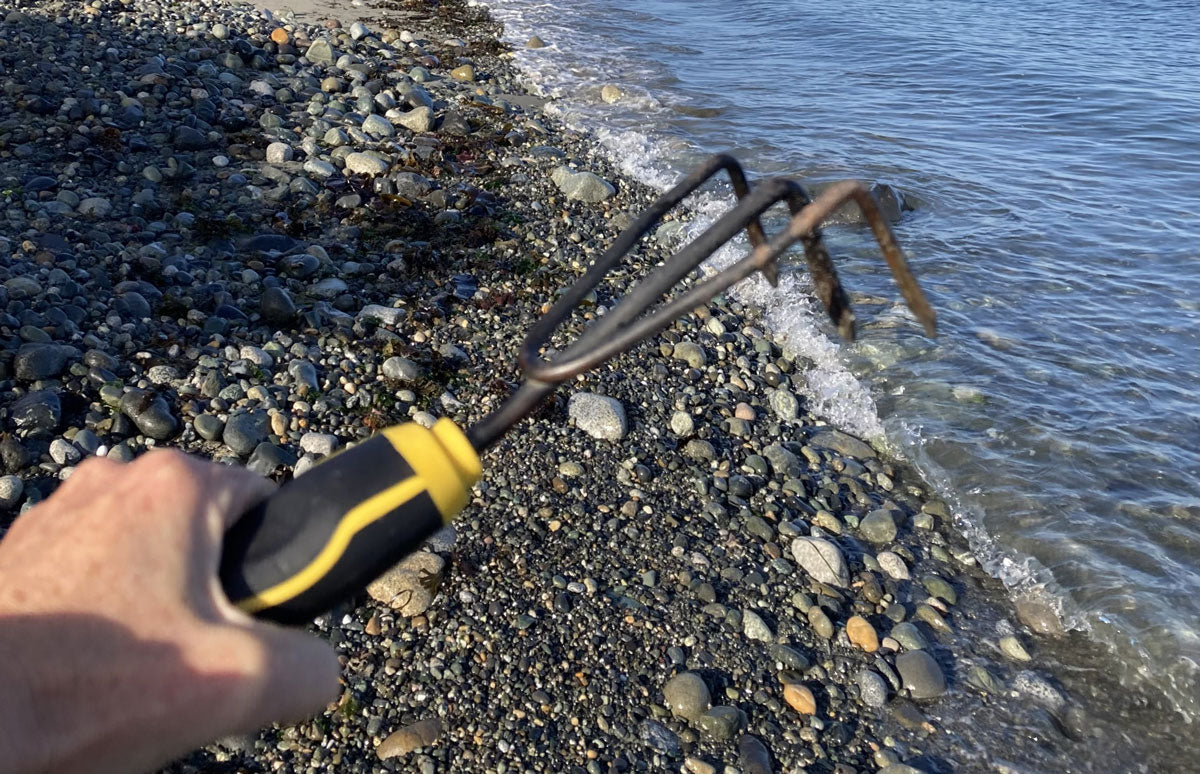A person stands on a rocky beach beside the water, holding a small, handheld garden rake in their left hand. The rake features a black and yellow handle and three short, rusty prongs that curve to a point. To the right, gentle waves wash onto the shore, which is covered with an assortment of smooth, rounded stones. The stones vary in shape and size; most are small and predominantly gray, with some exhibiting shades of green, orange, and white. Further from the water, larger, rounder rocks can be seen, creating a picturesque and textured shoreline.